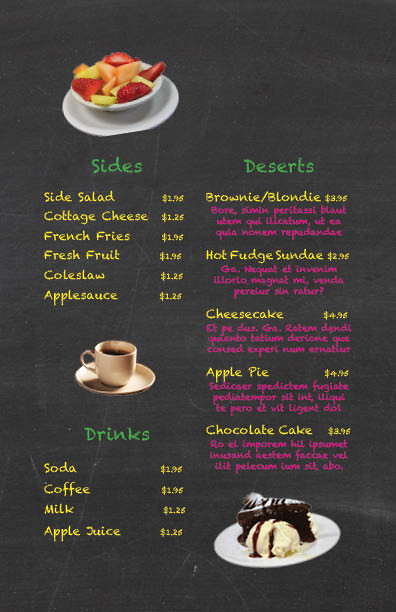Displayed is a detailed segment of a restaurant menu set against a black backdrop. The menu is divided into three primary sections, each highlighted with green text: "Sides," "Desserts," and "Drinks." 

**Sides**:
- A vibrant fruit salad image is shown above this section.
- Options listed:
  - Side Salad: $2.95
  - Cottage Cheese: $2.25
  - French Fries: $1.95
  - Fresh Fruit: $1.95
  - Coleslaw: $1.25
  - Applesauce: $1.25

**Desserts**:
- Below the desserts heading, nestled within the list, is a tempting image of a chocolate cake with chocolate frosting complemented by a scoop of vanilla ice cream.
- Choices available (highlighted in yellow):
  - Brownie/Blondie: $2.95
  - Hot Fudge Sundae: $2.95
  - Cheesecake: $4.95
  - Apple Pie: $4.95
  - Chocolate Cake: $1.95

**Drinks**:
- A rich cup of coffee is displayed above this section.
- Selections include:
  - Soda: $1.95
  - Coffee: $1.95
  - Milk: $1.25
  - Apple Juice: $1.25

The detailed, visually appealing arrangement of the menu items is both inviting and informative for potential diners.